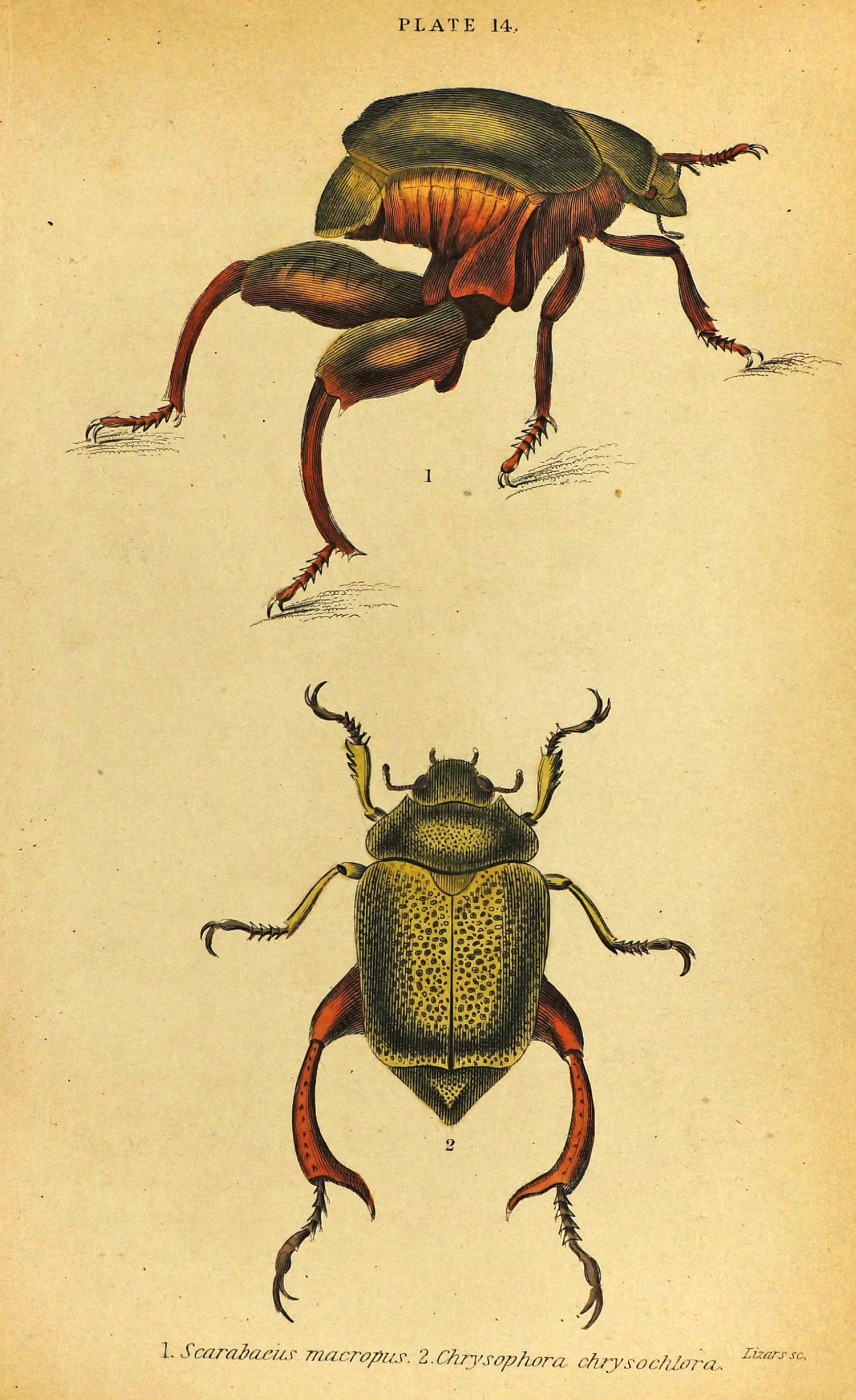The image depicts a detailed drawing of an insect on a light brown, yellowed paper, reminiscent of an old natural history book. The page is labeled "Plate 14" at the top center. The artwork includes two colored sketches of the same beetle from different angles – one at the top shows the insect in a walking position, viewed from its back and side, with its rear end pointed towards the bottom left and its head towards the bottom right. The other sketch at the bottom displays the beetle from a top-down perspective, with its head at the top, tail at the bottom, and legs extended outward.

The beetle has a green upper body adorned with black spots, while its lower body is primarily brown with a metallic, copper hue. It features six legs and two prominent antennae on its head. The detailed illustration captures slight lines on the head and a tapered shell on the back. Notably, the beetle's body is elevated significantly from its back legs.

At the bottom center of the page, the scientific names "Scarabuccus micropus" and "Chrysophora chrysocolora" are inscribed in black text, likely labeling the different orientations or possibly different species represented in the sketches.